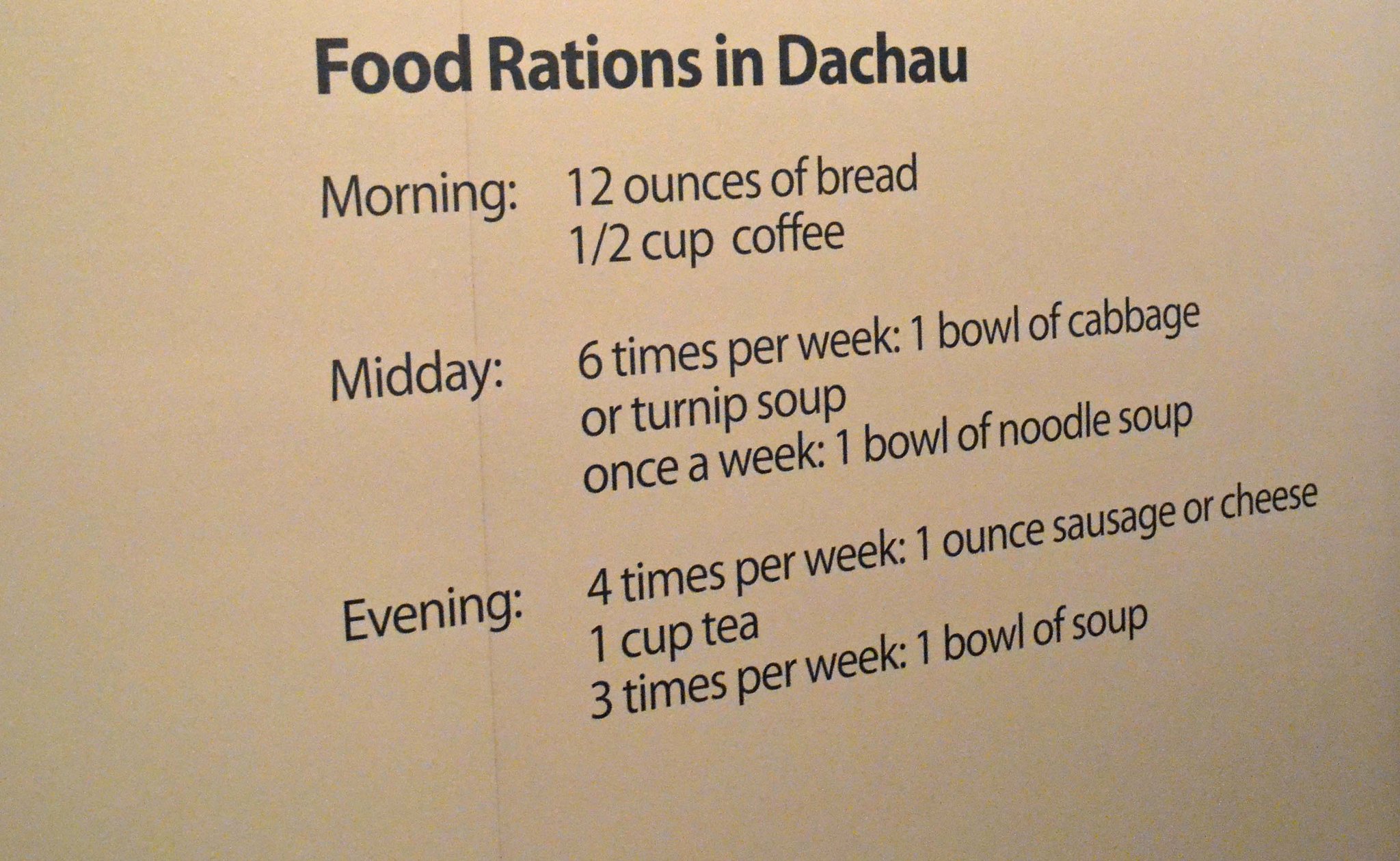This is an image of a light brown, horizontally oriented card displaying the food rations provided to prisoners in Dachau Concentration Camp. The card, printed with black text, outlines the dismal daily allotment of food. At the top, in bold, it reads “Food Rations in Dachau.” The morning ration consists of 12 ounces of bread and half a cup of coffee. For midday, six times per week, prisoners received one bowl of cabbage or turnip soup, with a bowl of noodle soup allocated once a week. In the evening, four times per week, the ration included one ounce of sausage or cheese and one cup of tea, with an additional bowl of soup provided three times per week. These minimal and inadequate rations were indicative of the brutal conditions designed to weaken and starve the inmates.